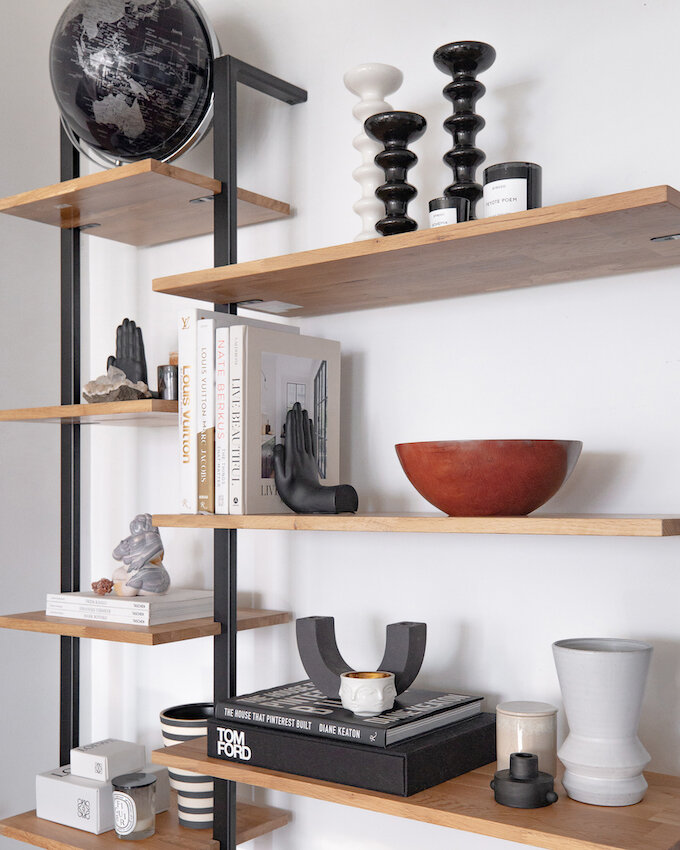This image features two columns of modern, minimalistic shelving against a white wall, showcasing a variety of decorative items. The shelving on the left is a four-tiered narrow unit supported by black metal posts, while the right side features a three-tiered, wider structure made from matching light-colored wood.

On the top shelf of the left unit sits a striking black globe with grey accents. Below it, a stylized black hand sculpture accompanies what appears to be a gemstone or geode. The third shelf holds a trio of white books with a small grey Buddha statue, and the bottom shelf displays two white boxes of varying sizes alongside a glass jar and a black-and-white striped cup.

The right-hand side shelves host a curated collection of similar aesthetic. The top shelf presents black and white candlestick holders along with two large jar candles. Below that, a red bowl is flanked by a hand-shaped bookend supporting several white books. The lowest shelf showcases two black books topped with a U-shaped piece of artwork and is accompanied by a white vase and a smaller, cream-colored vase. The objects on both sides include coffee table books with prominent logos like Louis Vuitton and Tom Ford, exuding a sense of fashionable sophistication. This arrangement highlights a blend of art, literature, and modern design, creating a prominent display likely intended as a focal point in a contemporary living space.